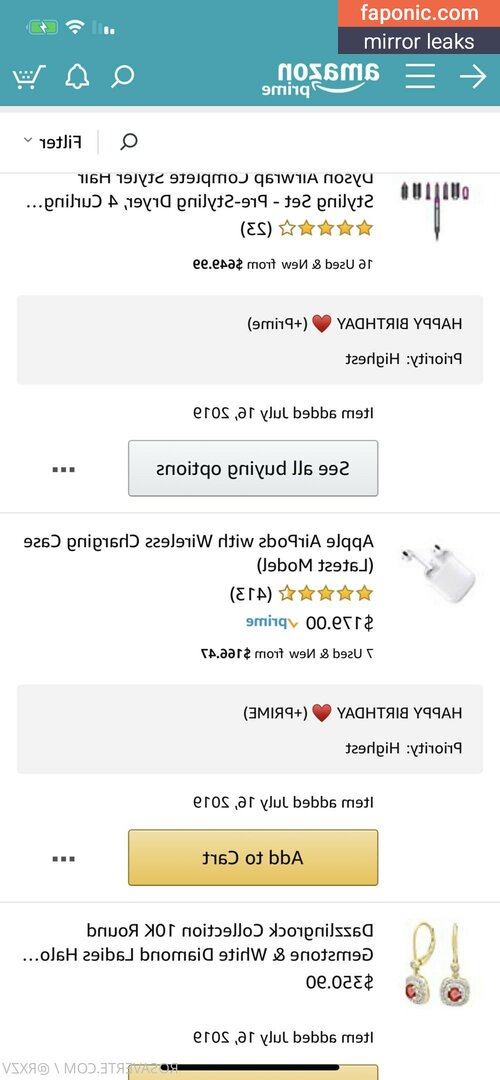A mirrored screenshot of the Amazon app taken on a mobile device displays various elements of the app's interface in reverse. In the top left corner, a battery icon with a lightning bolt indicates the device is charging, alongside cellular and Wi-Fi signal strength icons. The top right corner features the text "faponic.com mirror leaks." Below, the reversed Amazon Prime logo is visible, along with icons for the cart, notifications, and search functions. Underneath, the search bar includes a filter button. The displayed items begin with a Dyson product, likely the Dyson Airwrap, showing four stars next to its price. Below, listing Apple AirPods, rated at four and a half stars, includes the price and a Prime shipping logo. Further down, a pair of earrings is displayed with its corresponding price. The reversed text throughout the image makes it challenging to interpret, but the products and ratings are discernible.